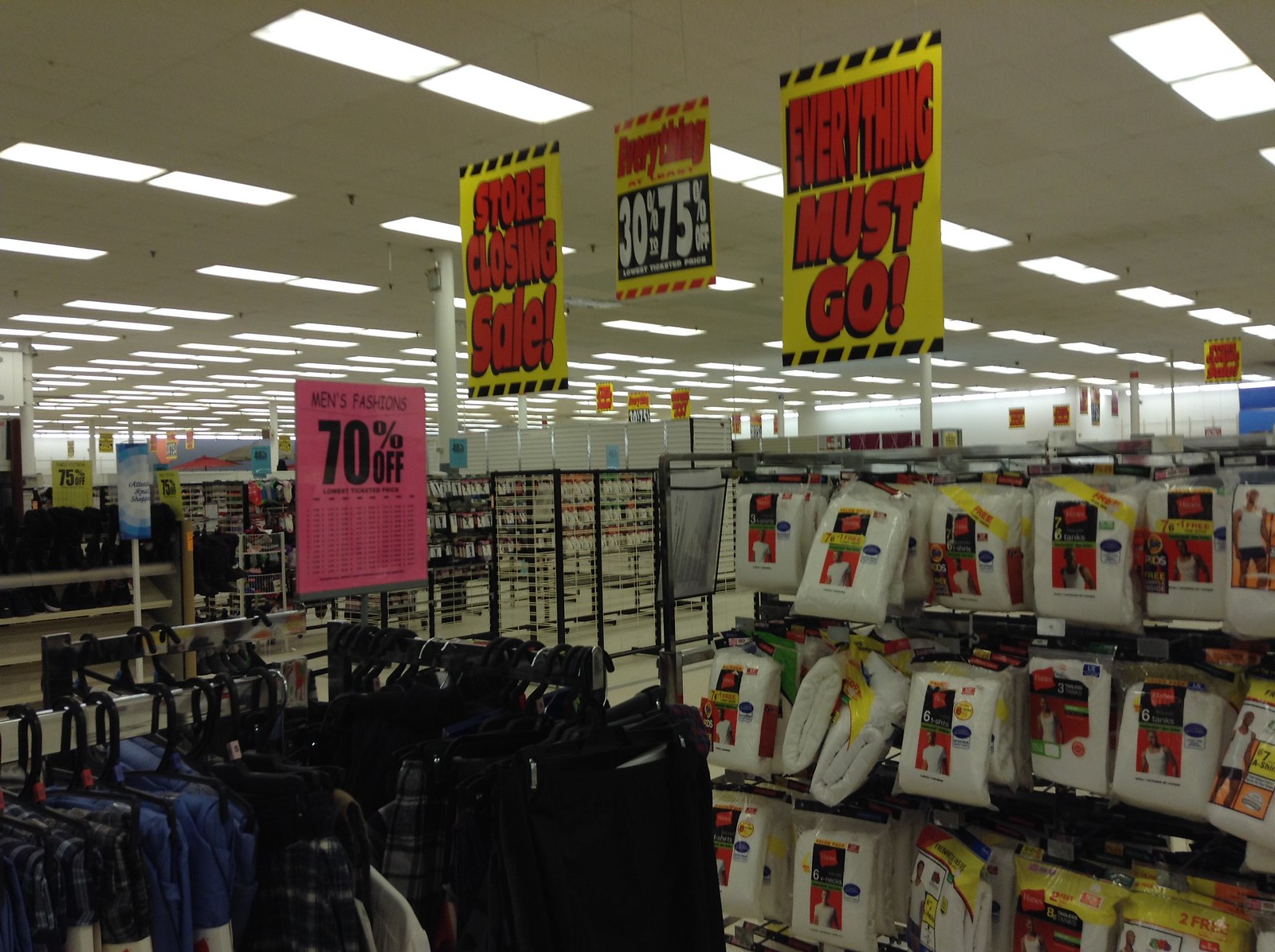The photograph captures the interior of a large variety store, currently undergoing a closing sale. The ceiling, fitted with recessed lighting and acoustical tiles, features overhead sprinklers. Banners, strung from wires suspended below the ceiling, prominently advertise significant discounts: "Foreclosing Sale," "70% Off," "Everything Must Go," and "30% to 75% Off."

The image focuses on the men's apparel section, showcasing garment racks filled with neatly arranged slacks, t-shirts, and briefs. In the background, the view extends to more clothing items, including underwear and socks. A distant sign reiterates the substantial markdowns with a bold "75% Off." The store is a quintessential example of a big box retailer in its final days, offering significant discounts as it prepares to close its doors.